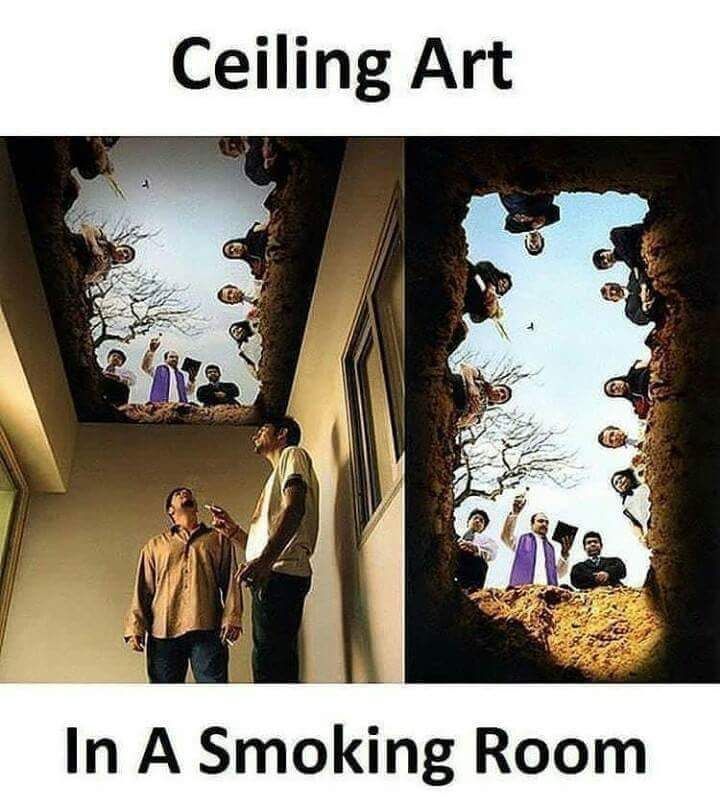The image is a thought-provoking composition split into two detailed photographs, with added text for context. The top of the image features the caption "ceiling art" in black letters, while the bottom reads "in a smoking room." On the left side, there are two men standing in a room with tan-colored walls; both are smoking cigarettes, and one is looking upwards. The ceiling above them has an open hole. Within this hole, a scene is depicted, showing a group of people huddled around, visible as if looking down from above. A religious figure, identifiable by a purple stole and holding a book, appears to be performing a ceremonial reading. Surrounding the hole are tree branches and a blue sky, indicating an outdoor setting beyond the indoor space. The right side of the image provides a close-up of this ceiling art, emphasizing the mournful gathering around what represents a grave. This symbolizes the smoker as the person in the grave, blending the smoking room's ambiance with the visual of mortality and remembrance. The overall color palette includes black, white, light blue, brown, tan, purple, and maroon, enhancing the scene's somber yet reflective tone.